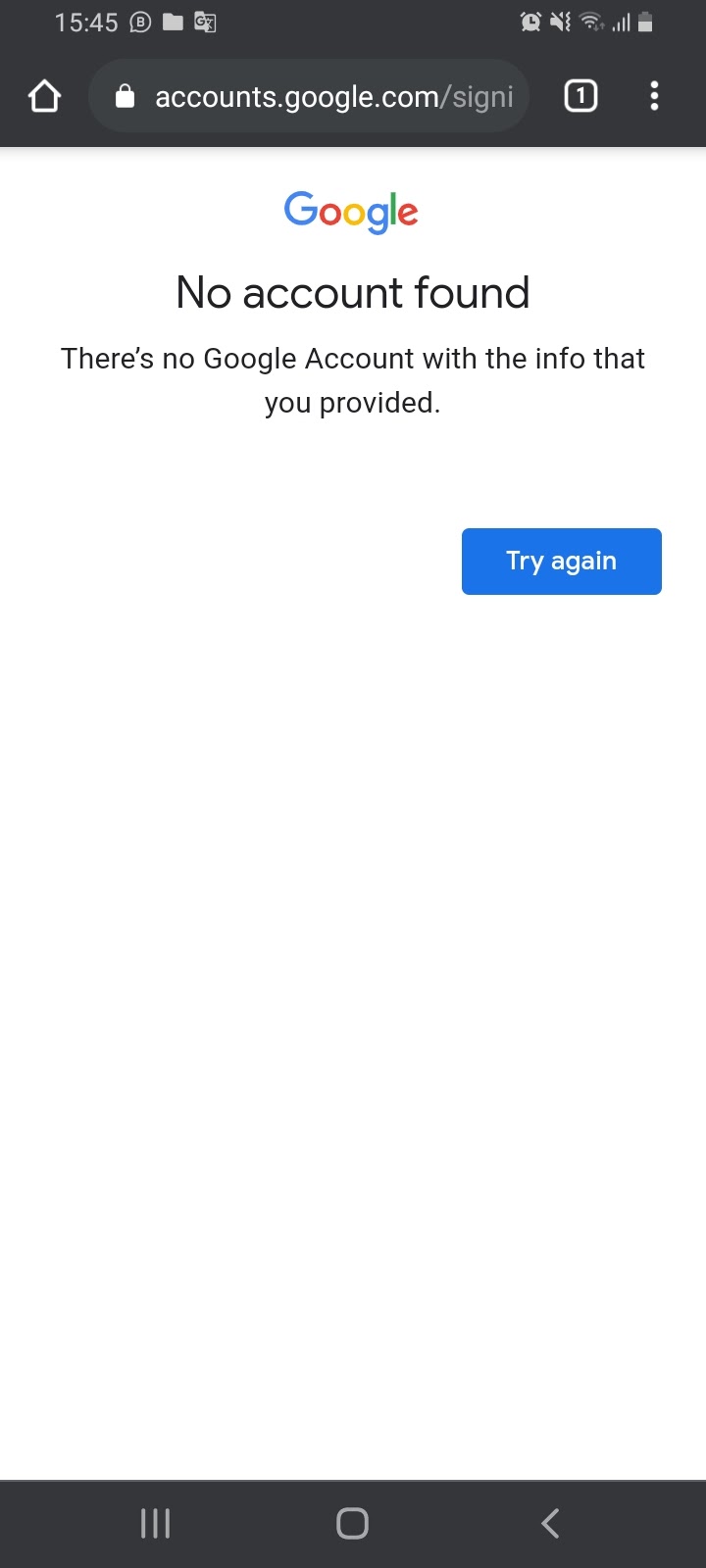The screenshot from the phone displays various elements arranged on a screen, described in detail as follows:

At the top, there is a black rectangle information bar. In white text, the time is displayed as 15:45. Next to the time, there is an icon with a 'B' symbol, followed by a file folder icon, and then another unrecognized icon. Moving to the right within the black bar, there are several icons in sequence: a clock, a speaker icon with a slash through it indicating muted sound, a Wi-Fi signal icon, cellular bars, and a battery icon showing approximately two-thirds remaining charge.

Beneath this black bar, there is an icon of a house, followed by another black space, and an icon of a lock. This lock icon is situated within a lighter, rounded rectangle. Next to the lock icon, the text reads "accounts.google.com," followed by a grayed-out slash and the partially visible text "sign" (S-I-G-N-I). To the right, there is a white square within a black background containing the numeral '1', followed by another black space and vertical three dots menu icon.

Below this information, the colorful Google logo is displayed with the text "No account found" underneath. A subsequent line of text states, "There is no Google account with the info that you provided." After a triple space, the screen suggests, "Try again." The rest of the screen remains blank until reaching the bottom border, which features three icons.

This detailed description encapsulates the entirety of the phone screen's visible elements and their respective placements.